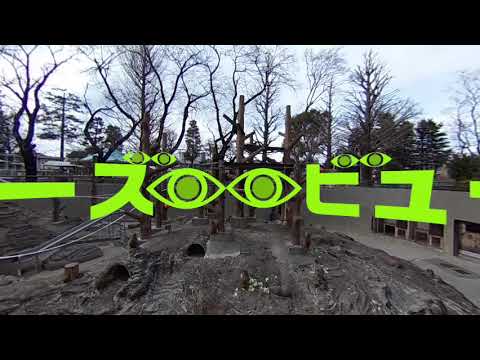The image depicts an outdoor scene dominated by a vibrant lime green hue, likely suggesting some kind of themed event or immersive environment, potentially inspired by an Asian aesthetic given the presence of Asian characters. The background features a light blue sky dappled with dark gray clouds, casting a muted daylight over the setting. 

Various trees populate the scene, with many bearing bare, lanky branches, although a few pine trees retain their foliage. The ground is predominantly gray, covered in dirt with visible trenches and burrowed tunnels, suggesting significant human or natural activity.

Central to the image is a large wood-crafted structure, resembling a chair made from cut tree limbs, reinforced by a ramp and railings leading to an assortment of logs and bridges, potentially indicative of an obstacle course. To the right, a stone wall adorned with multiple glass doors and windows provides a stark, modern contrast to the natural elements.

Additionally, a scattering of flowers can be seen amidst the otherwise earthy tones, enlivening the scene. Prominently placed are graphics of three pairs of neon green eyeballs, contributing to the surreal atmosphere. In the distance, several eye logos further accentuate the scene, contributing to a coherent and immersive visual narrative.